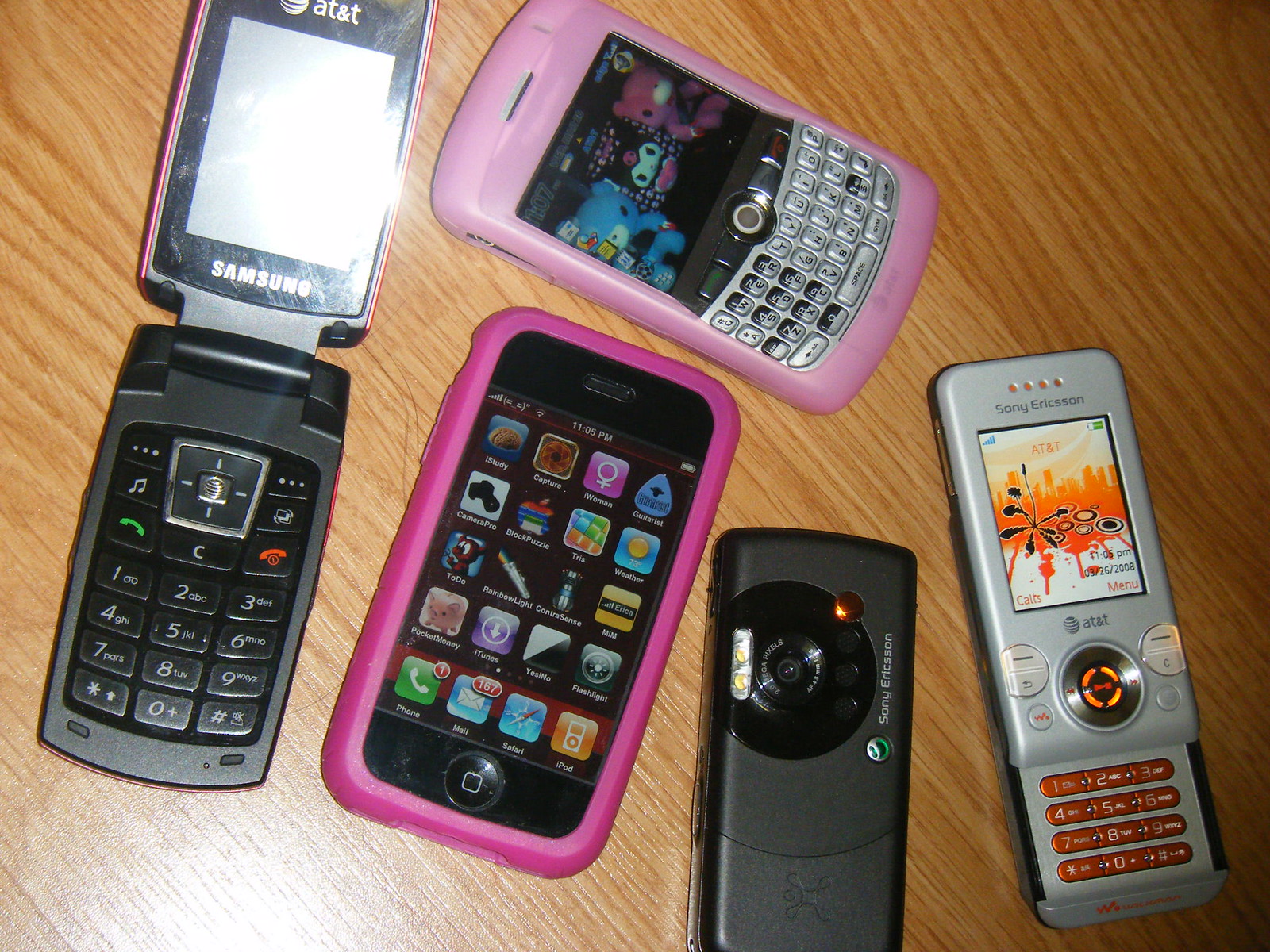This image displays six outdated cell phones arranged on a wooden table, reminiscent of a listing on eBay. From left to right, the phones include a black or dark gray AT&T Samsung flip phone, a first-generation iPhone in a hot pink case, and a BlackBerry adorned with a light pink case. Next to the BlackBerry is an unidentified phone showing only its back with a camera, and then a white Sony Ericsson slide phone, distinguishable by its orange-outlined keys. Finally, another unidentified Sony Ericsson phone is positioned as well. This collection exemplifies a variety of cell phone styles from the late 1990s to the early 2000s.